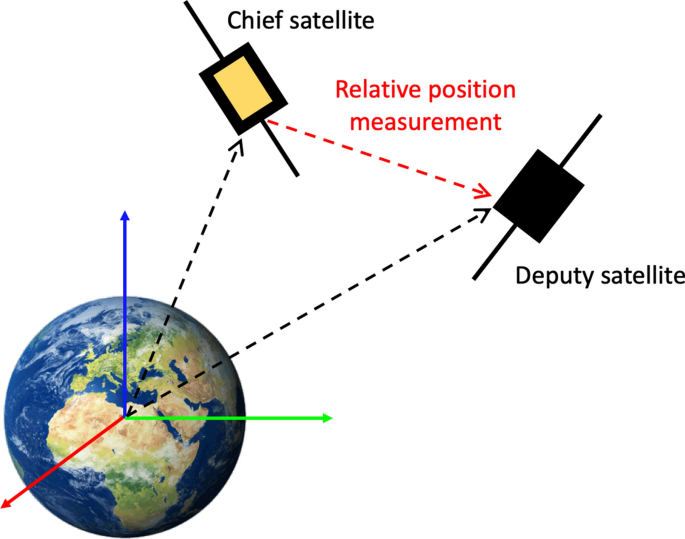The image depicts a detailed diagram set against a white background. In the bottom left corner, there is a 3D representation of Earth, vividly showing Africa in brown, yellow, and green hues, along with the ocean and some clouds. Three colored arrows represent different axes: a blue arrow pointing upwards, a red arrow pointing diagonally, and a green arrow pointing horizontally to the right. These arrows connect to two satellites depicted on the right side of the image. The Chief Satellite is shown as a black rectangle with a yellow center and lines indicating its position, and a similar black rectangle represents the Deputy Satellite. Dotted lines with arrows connect these satellites, with a prominent red arrow labeled "Relative Position Measurement" stretching between the Chief Satellite and the Deputy Satellite. Additional dotted arrows trace the connection from Earth to these satellites, elucidating their relative positions and coordinated measurements.